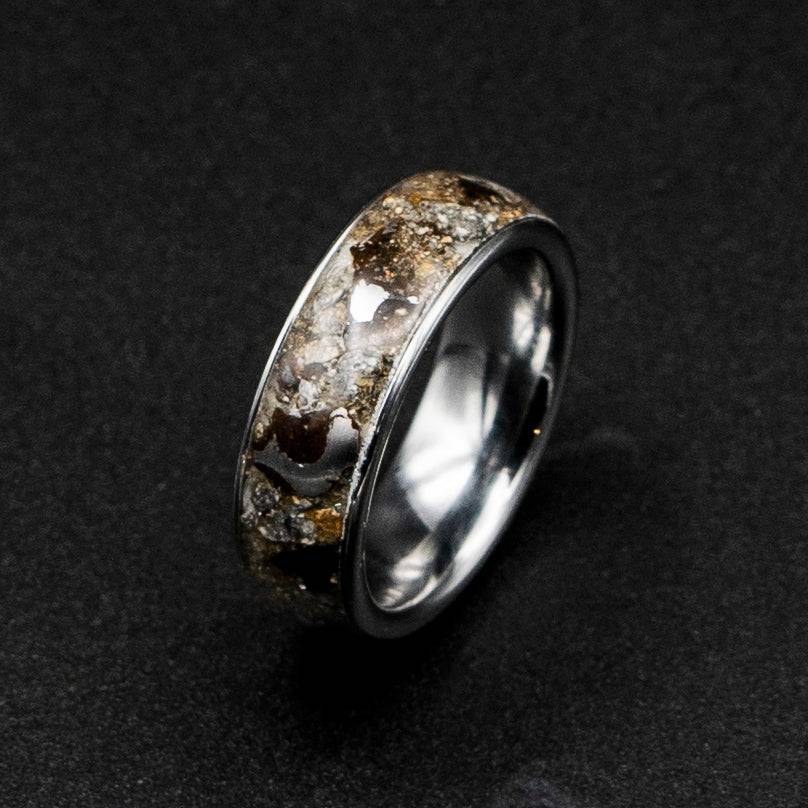The image showcases a detailed and elaborate ring prominently standing on its end. The ring features a shiny, silver inner core that catches the light and reflects brilliantly, creating a luxurious feel. The outer band of the ring is adorned with a granite-style design, characterized by an array of sparkly brown and gray hues dispersed in a random, non-pattern manner. This thick, masculine-design ring exudes an air of antiquity, suggesting it might be somewhat outdated but still finely crafted. Although the interior lacks engravings or markings, the careful placement of small gemstones on the exterior highlights the jeweler's meticulous attention to detail and intent to create a piece fit for royalty. The background of the image consists of dark charcoal gray, black, and shades of gray, possibly resembling a close-up of foam or fabric, providing a contrasting backdrop that further accentuates the ring's grandeur.